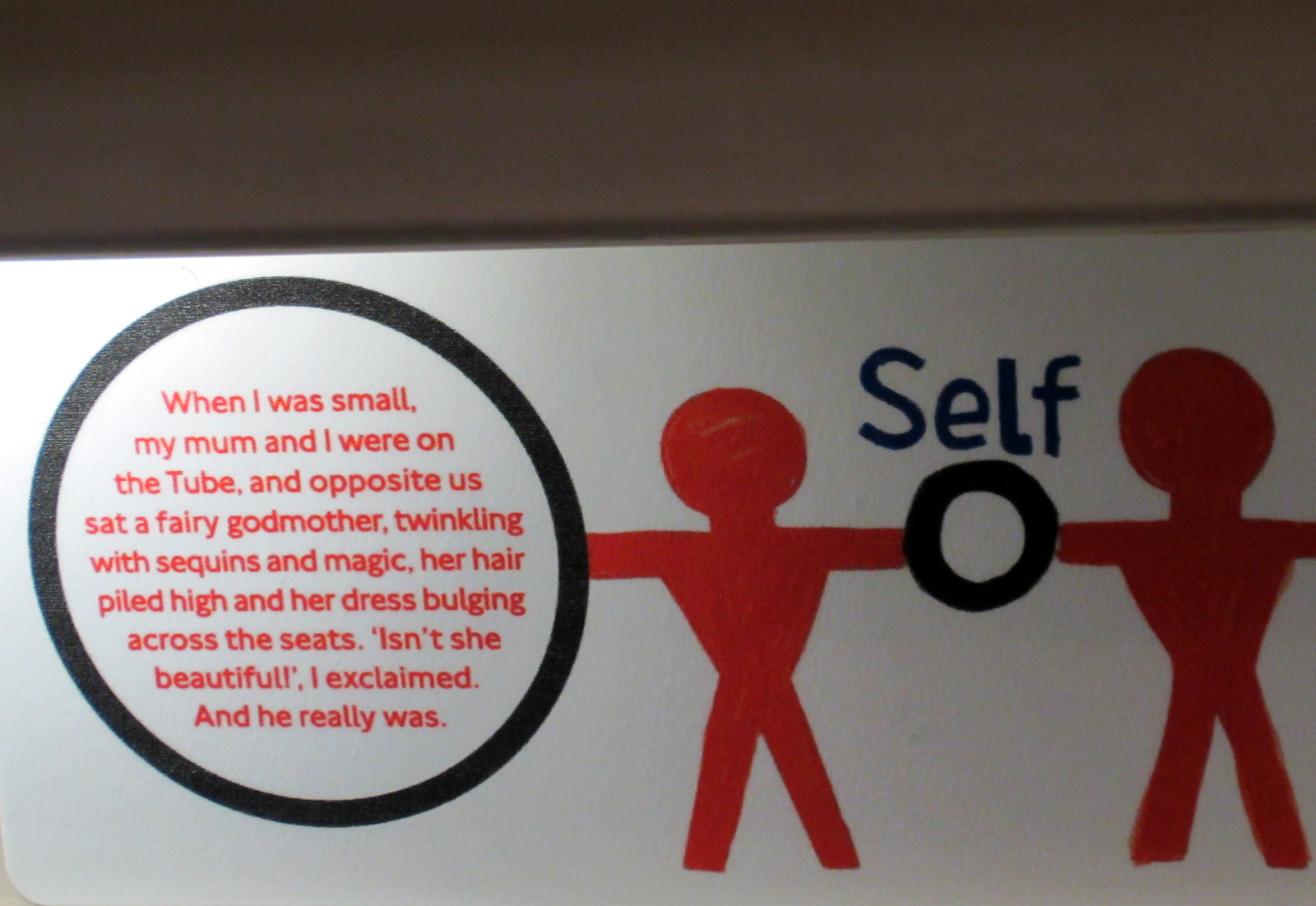The image depicts a wide, rectangular sign resting on a somewhat off-white surface, positioned close to the top of the frame and extending horizontally. The background is a dark gray wall, creating a small shadow where the sign meets it. Central to the image are two red stick figures with outstretched arms, positioned in such a way that their arms form a partial circle around a smaller black circle. Above this, the word "self" is written in black text. To the left of the leftmost figure, there is a larger black circle containing red text that reads: "When I was small, my mom and I were on the tube and opposite us sat a fairy godmother twinkling with sequins and magic, her hair piled high and her dress bulging across the seats. 'Isn't she beautiful?' I exclaimed, and he really was." The sign overall stands out against the darker, plain gray background of the wall behind it.